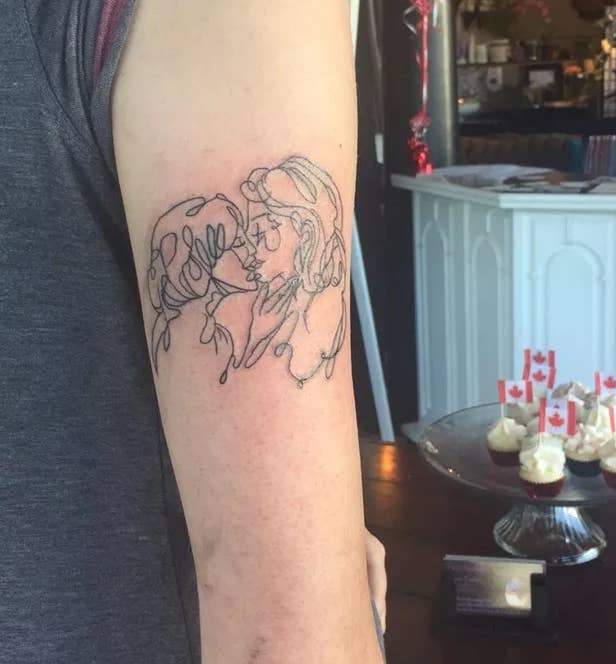The image depicts a recently done tattoo on a person's upper arm, showcased in a color photograph with a square format. The tattoo, located on the outside of the upper arm, extends from the top of the shoulder to just below the elbow and features two women kissing, depicted in profile with their lips touching. The design is created using curvy, continuous lines that swirl and form the side profiles of the women, one with shorter hair and the other with longer hair. The skin around the tattoo appears pink and inflamed, indicative of its recent application. The background includes a crystal platter with cupcakes adorned with white frosting and small Canadian flags, a white cabinet, and barware positioned above. The tattoo fills most of the arm's horizontal space and employs a style blending representationalism with artistic line work.